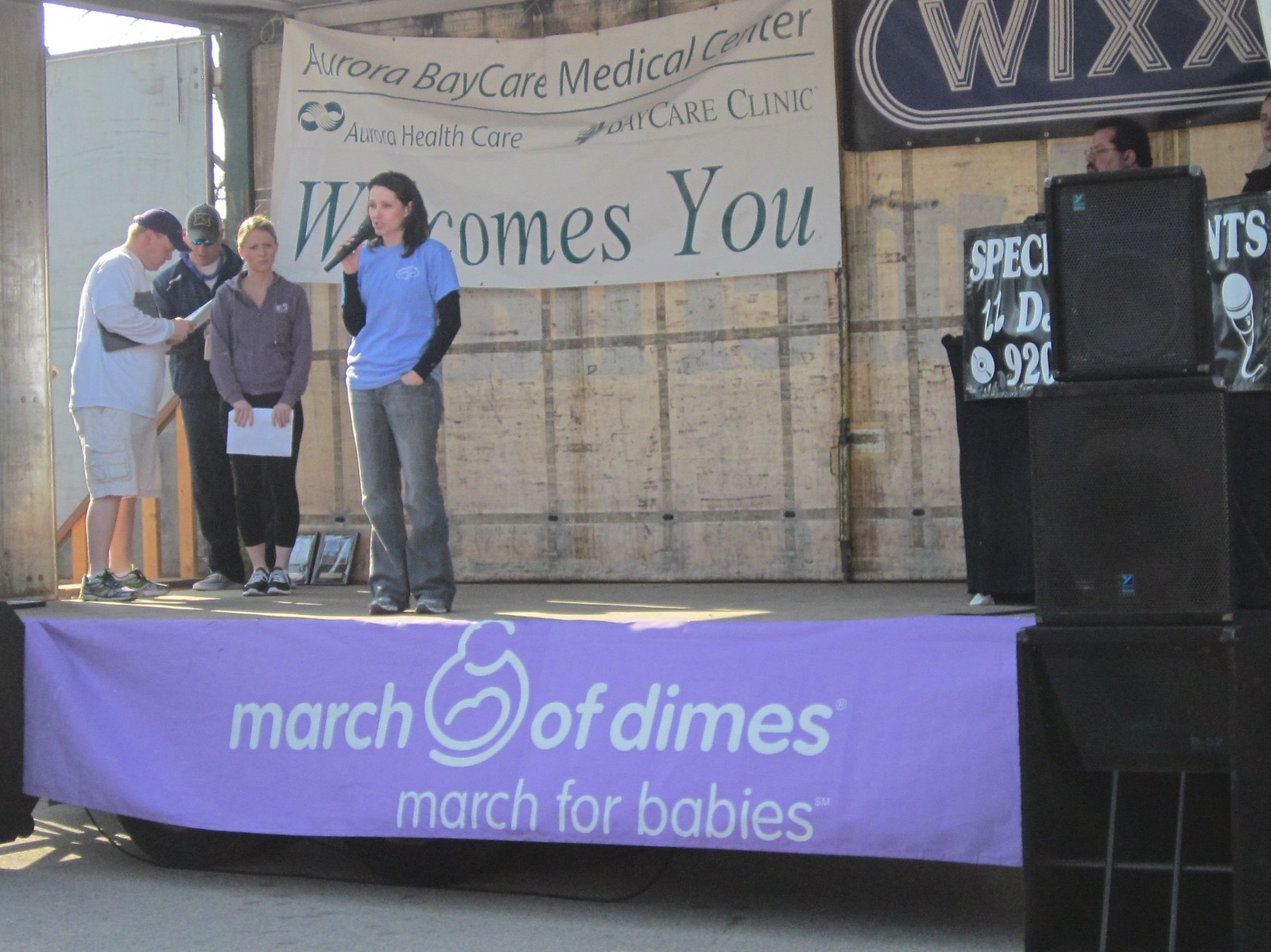The photograph captures an outdoor event featuring a small stage adorned with various banners and signs. At the forefront of the stage, a purple banner with white lettering displays "March of Dimes, March for Babies," accompanied by a graphic of a woman holding a baby. Behind the stage hangs a large white sign with green font, reading "Aurora BayCare Medical Center, Aurora Health Care and BayCare Clinic welcomes you." To the right of this banner, a black sign with gold lettering indicates "WIXX."

On the stage, a woman with black hair, dressed in a light blue short-sleeved shirt over a long-sleeved black shirt and gray pants, speaks into a wireless microphone. She stands confident, addressing the audience. Beside her, to the right, another woman holds papers and watches attentively. Two men are engaged in a conversation behind her, occasionally glancing at the speaking woman.

To the far right of the stage, three speakers are stacked on top of each other, partially obscuring a background figure, whose head peeks out from behind the speakers. Overall, the image captures a moment of engagement and interaction during a community event.